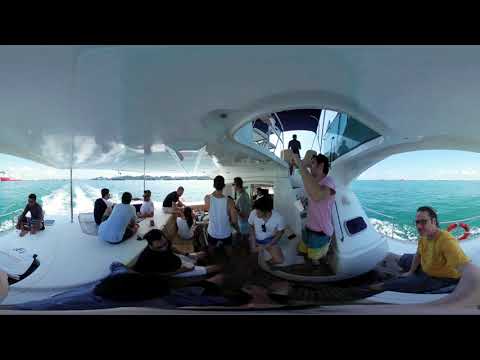A vibrant scene on a modern two-level yacht captured with a fisheye lens, creating a panoramic, wraparound effect. Around 15 to 20 people are aboard, dressed in breezy beachwear featuring pinks, whites, and yellows, clearly enjoying a sunny day on the water. On the far left, you can see the greenish water splashing behind the moving boat, trailing bright white foam. The bottom deck hosts most of the passengers, who are sitting and chatting comfortably on benches that border the edges of the boat. A man in a black shirt sits at the far left edge near a thin white barrier, while nearby another person, seen from behind and dressed in a red and white shirt, converses with a person in a black shirt. Central to the image is a jubilant figure in a pink shirt and blue and yellow shorts, arms raised in joy. On the far right, a man in a white shirt and blue pants, sunglasses on and hair neatly combed back, leans forward slightly. Behind him, the bright greenish ocean extends to the horizon. The top deck is accessible via a stairway and features another individual, visible in black silhouette against a white and black interior. The overall ambiance suggests a lively party atmosphere with people socializing and relishing their picturesque maritime excursion. In the far background, there's a reddish boat and distant landmass, adding depth to this idyllic seascape.